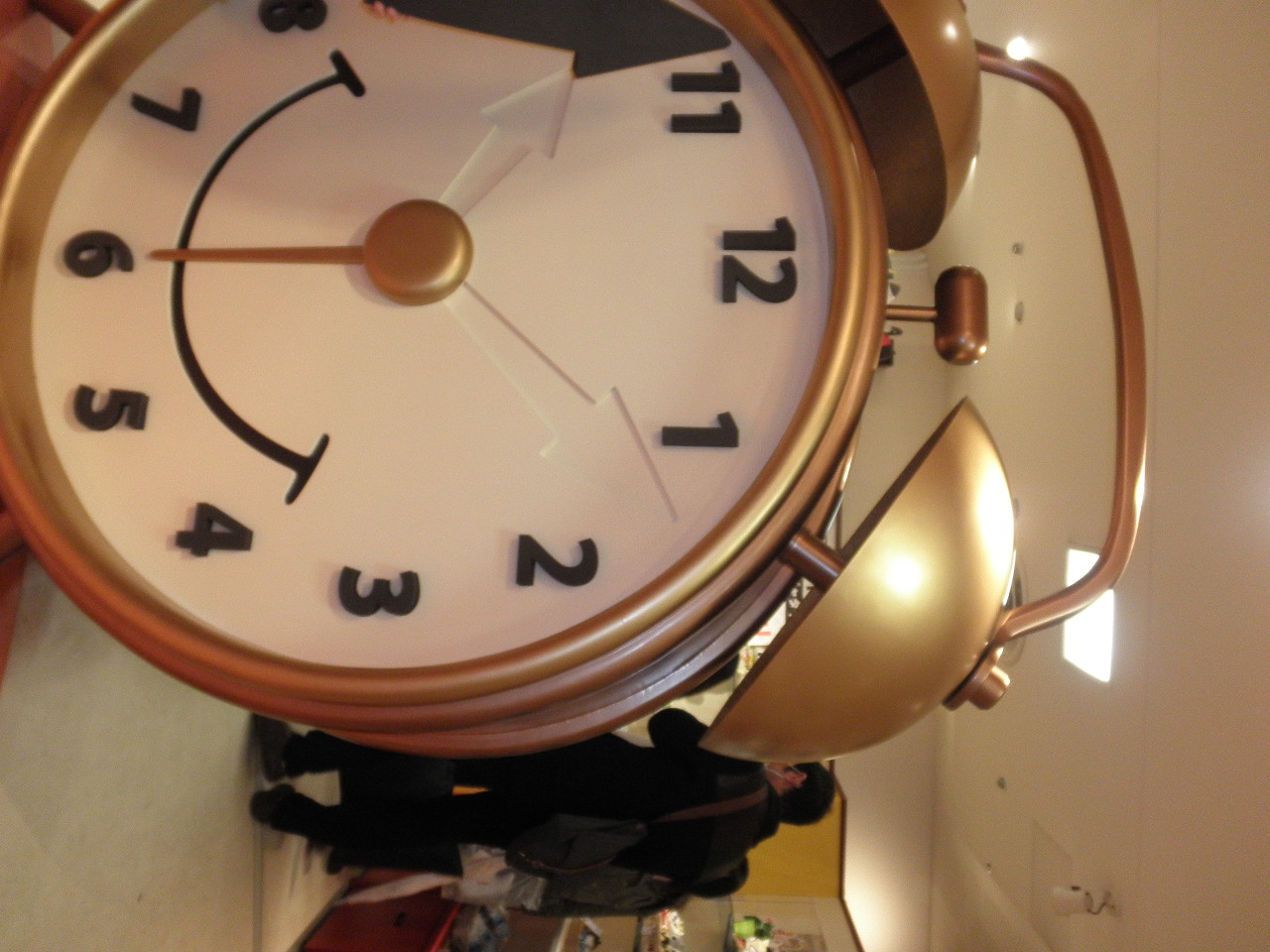In this image, an old-fashioned brass double bell alarm clock prominently takes center stage in the foreground. The clock features a classic design with two brass-colored bells positioned at 1 o'clock and 11 o'clock, connected by a brass bar with a hammer resembling a mallet poised to strike them. The clock's housing is also brass, complementing the bells. Its face is a stark white, contrasting with the black numerical markings. Notably, the hour and minute hands are missing, leaving only a loose hand positioned between 8 and 11, lying sideways. A large gold knob at the bottom center, with a needle-like indicator pointing to 6 o'clock, is marked by a smiley face-like curve extending from 8 to 4, hinting at the clock's non-functional or whimsical nature, possibly suggesting it might be a display item or a toy rather than a functional timepiece.

In the background, a room with a low wall lined with shelves is visible. The shelves host various items, though details remain indistinct. To the center-right of the image, a gentleman stands with his back to the camera, dressed in a dark jacket and dark-colored pants. Beside him, another figure with dark hair, also clad in a dark-colored jacket and matching slacks, stands, partially obscured. The overall scene combines elements of nostalgia and mystery, anchored by the detailed depiction of the unique alarm clock.